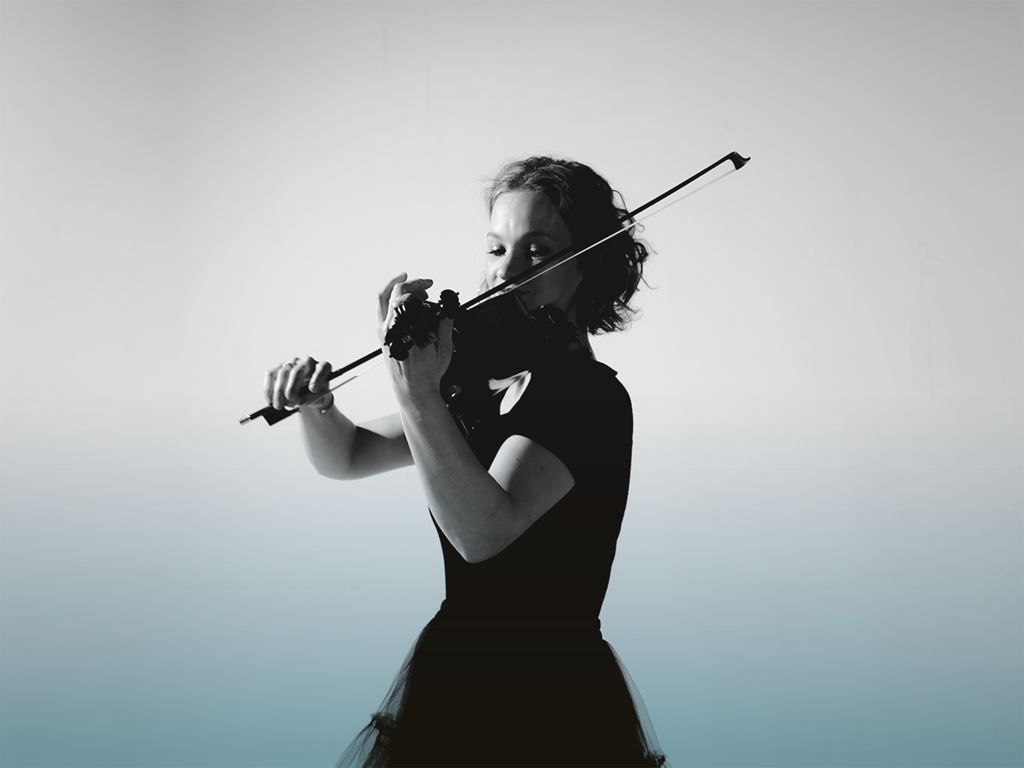This is a square black and white image featuring a woman playing the violin against a plain background that transitions from light gray at the top to light blue at the bottom. The woman has short, possibly light brown or dark blonde hair with a slight curl at the back. She is captured from her left side, both elbows bent as she holds the violin with her left hand and chin, while her right hand expertly strokes the bow across the strings. She is dressed in a black outfit, consisting of a black dress with lace details on the front and back, and a short-sleeved top. The image is cropped above her thigh, focusing on her poised and confident stance as she looks down at her instrument, indicating her deep concentration and likely extensive experience in playing the violin.